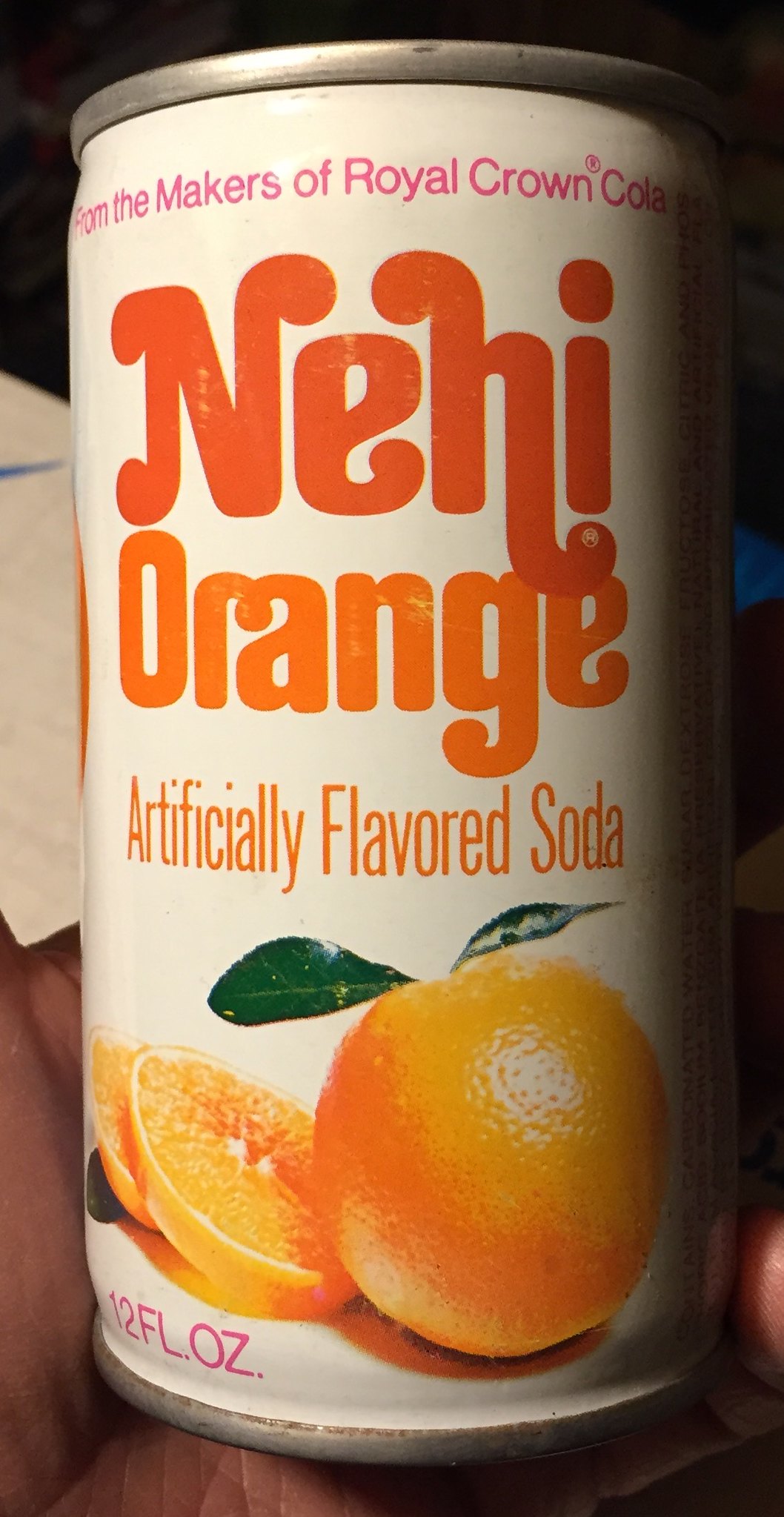The photograph captures a vintage can of Nehi Orange artificially flavored soda, prominently displayed against a starkly contrasted background. The can has a white backdrop with a silver rim at both the top and bottom edges. At the very top of the can, purple text reads, "From the Makers of Royal Crown Cola." Below this in orange, the name "Nehi" is spelled out in a darker shade, with the word "Orange" underneath in a lighter hue. Smaller orange text beneath this states "Artificially Flavored Soda." The central graphics feature two oranges: one whole, adorned with dark green leaves, and the other sliced in half. At the very bottom, it reads "12 FL OZ" in purple letters. The image shows a Caucasian hand holding the can from the bottom, with fingers just visible on the left, bottom, and right sides of the frame. The background is dark on the upper left and right, with a whitish area near the center and a hint of dark blue in one corner. The image has a classic, almost nostalgic feel, suggesting the can could be a design from an earlier time period.